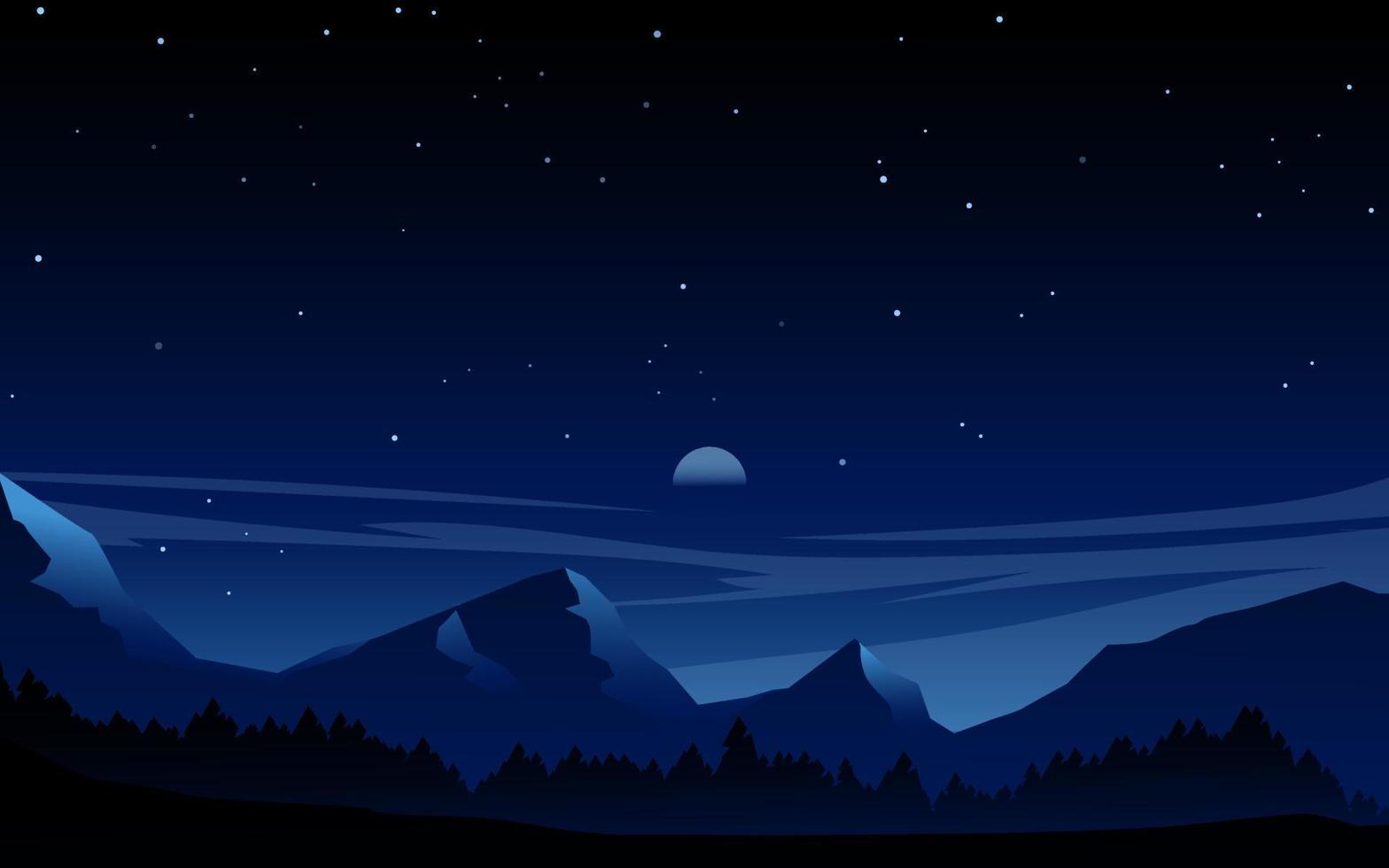The image is a digital drawing of a serene nighttime landscape. The sky transitions from a dark navy blue at the top to a lighter blue as it descends, with wisps of light blue clouds scattered throughout. White stars of various sizes are sprinkled across the sky, adding a tranquil, peaceful feel to the scene. The moon, half-visible and round, is a soft blue-white hue, hanging subtly in the background. Below the celestial display, jagged peaks of dark blue mountains rise, creating a rugged terrain. The bottom part of the image features the silhouettes of trees, their black outlines stark against the blue backdrop, giving the impression of a dense forest. The scene captures the stillness and calm of a starry night in the great outdoors.